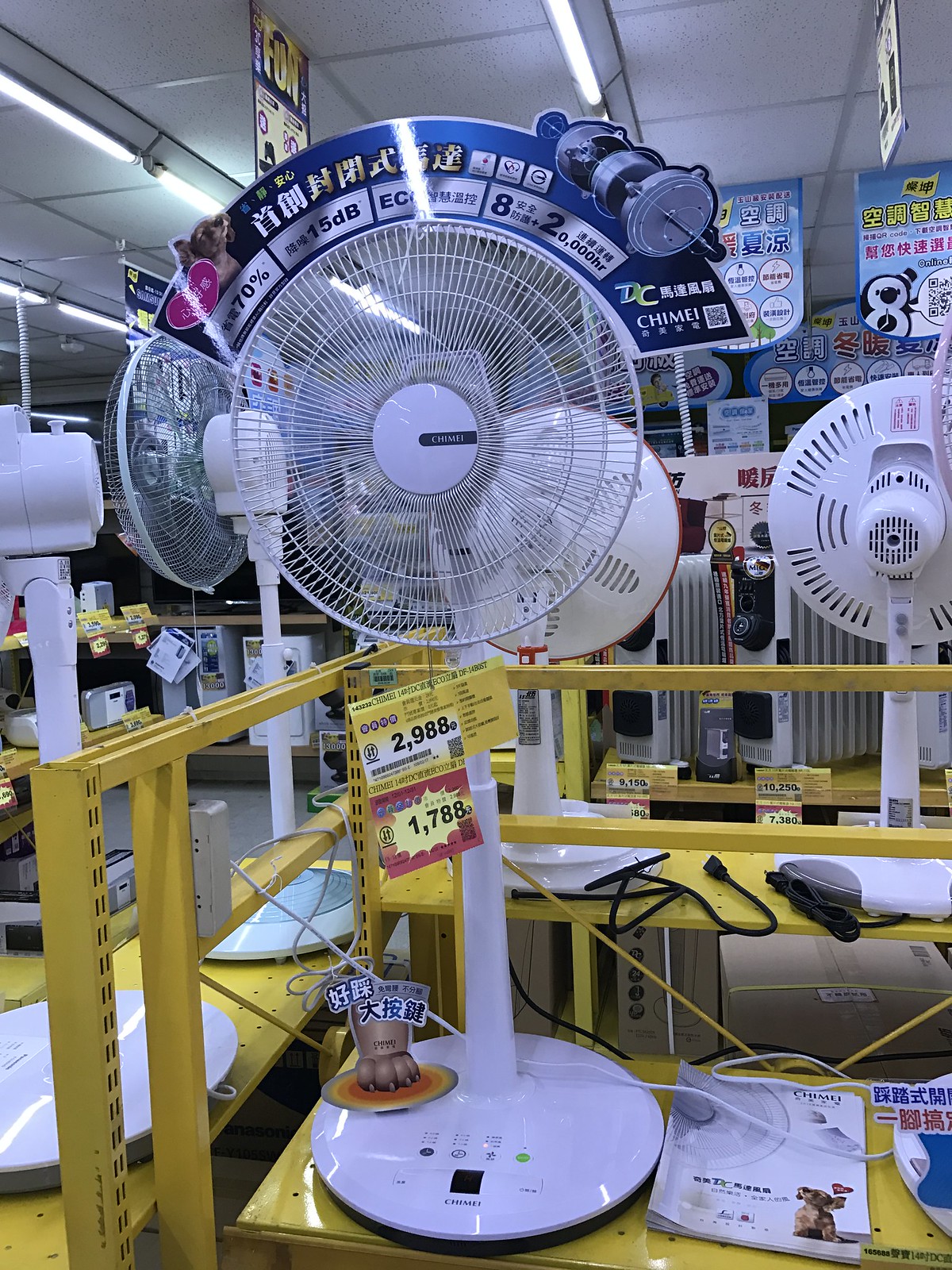The image depicts a vibrant scene inside a specialized store dedicated to selling fans and air conditioners, with a clear emphasis on a prominent sales display. At the forefront, a sturdy yellow steel rack holds a large white pedestal-type oscillating fan, which is turned on and running. The fan stands on a sizable circular base, which has an instruction booklet lying flat to its right. Dangling from the apex of the fan are two distinct price tags: a yellow and red tag displaying the original price of ¥2,988, and a red tag with a yellow starburst indicating a sale price of ¥1,788. 

The fan is branded "Chimei," highlighted with an advertising sheet that includes Japanese characters and specifications like "70%", "15 DB," and "20,000 hours." Surrounding this central fan are several other fans arranged around the edges of the yellow rack. To the left, more fans can be seen beyond a yellow steel rail. 

In the background, the store features long fluorescent light bulbs mounted on a white ceiling, adding brightness to the scene. There are also various banner signs hanging from the ceiling adorned with Asian fonts and colors, including blue with white letters and yellow and red lettering, though the exact text is unreadable. Additionally, the bottom shelf beneath the fan features some small signs, a gold figure, and a couple of magazines, one with a white cover and another with a blue and red design. The entire setup is neatly organised within the yellow metal fencing, enhancing the focus on the merchandise displayed.